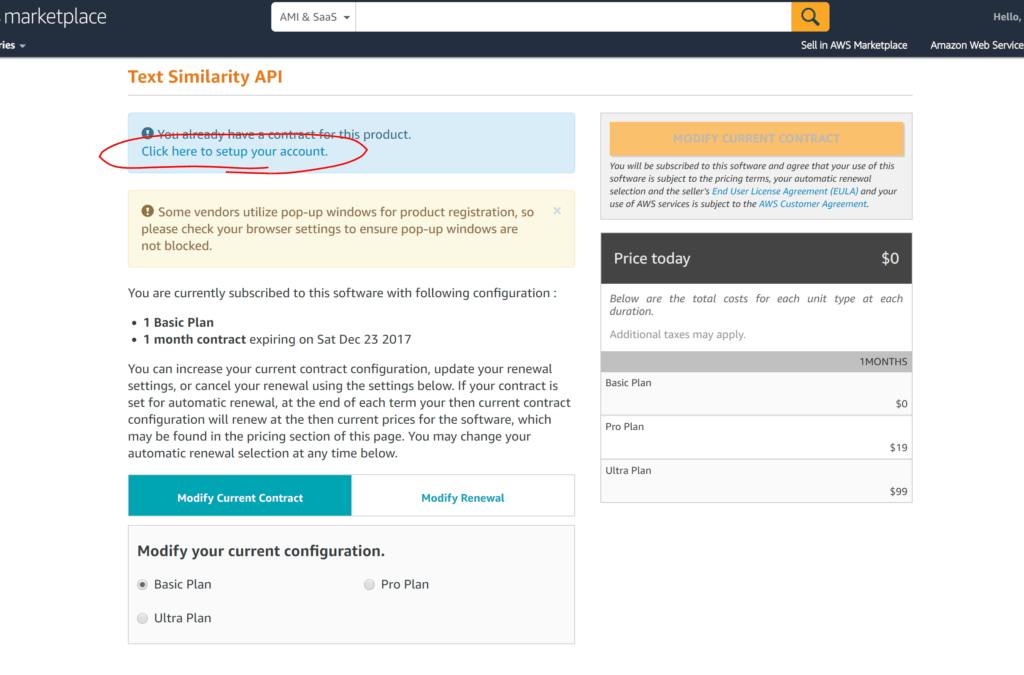This image is a screenshot from a website’s page for a text similarity API. At the top, the navigation bar reads "Marketplace," and contains a search area with placeholders “AMI” and “SAAS”. Below this, there is a white search bar with an orange magnifying glass icon on the right that serves as a clickable button for search functionality. 

Prominently displayed in bold orange text is the label “Text Similarity API.” Below this, a notification states, "You already have a contract for this product." Additionally, there is a clickable link, “click here to set up your account,” which has been highlighted with a red circle for emphasis.

Further down, a light yellow box contains a cautionary note: "Some vendors utilize pop-up windows for product registration, so please check your browser settings to ensure pop-up windows are not blocked." 

Continuing lower on the page, a subscription status section explains, "You are currently subscribed to this software with the following configuration:" followed by a bullet point list detailing a "Basic Plan" and a "One month contract," which is noted to expire on “Saturday, December 23, 2017.” Further information continues below this section, providing additional subscription details.